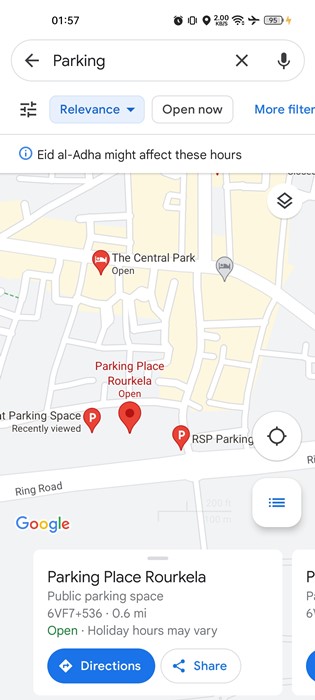The image displays a smartphone screen that is open to a maps application at 1:57 PM. The battery level is at 95%. The screen shows a search for nearby parking areas with filters set to "Relevance" and "Open Now." An alert at the top mentions Eid al-Adha, noting that it may affect business hours.

The displayed map highlights various locations, including Central Park and a parking place in Rukola. The app appears to be from Google, indicated by the familiar interface. The map pinpoints are marked in red, with some areas highlighted in yellow against a gray background. 

Nearby parking options listed include the "Parking Place Rukola," which is 0.6 miles away. There is a note that the place is open but advises that holiday hours may vary, potentially related to the Eid al-Adha warning.

The screen also features options to get directions, share the location, and access a menu through a hamburger icon, which suggests additional functionalities and filters.